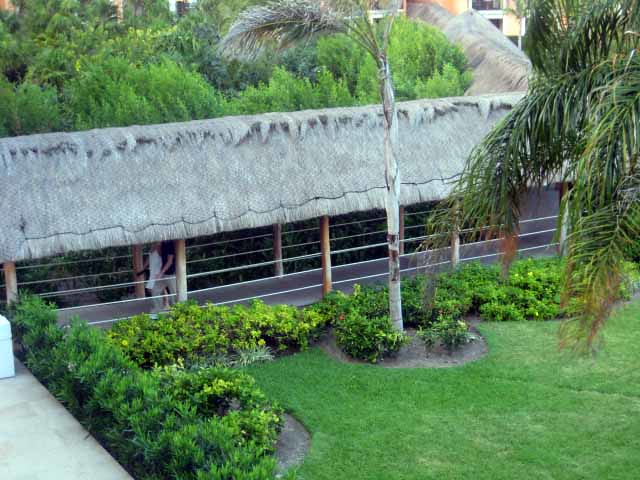The image depicts a well-maintained yard adjacent to a large building, featuring a hall-like section that people can walk through. This section is separated by a white string rail underneath a rather long gray roof and stretches from the left to the right, continuing towards the center. On the right side of the walkway is a manicured garden area with green bushes and a tree, while the top left corner of the image shows multiple very green trees and bushes. The walking path, which resembles a sidewalk, leads up to the building. The building itself has what appears to be a thatched roof and encircles a courtyard, creating a square shape. Various trees and plants extend over the roof, and a taller building is visible in the background. The garden also appears to have small yellow flowers among the greenery.